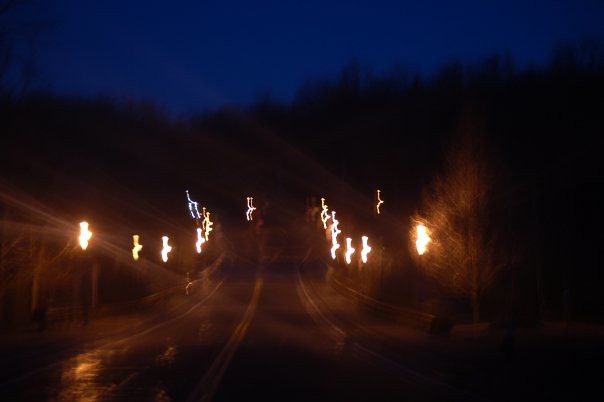A night-time photograph capturing a moonlit scene. The upper portion showcases a deep, dark blue sky, almost black, highlighting the silhouettes of tree tops beneath. The trees form a stark silhouette against the sky, rendering them nearly pitch-black. In the middle of the image, a road with two lanes is visible, marked by a yellow stripe running down its center, which glistens slightly, suggesting it might be wet. On either side of the road, a fence stretches out, illuminated intermittently by evenly spaced lights that fade into the blurry background, contributing to the depth and mystery of the night scene.